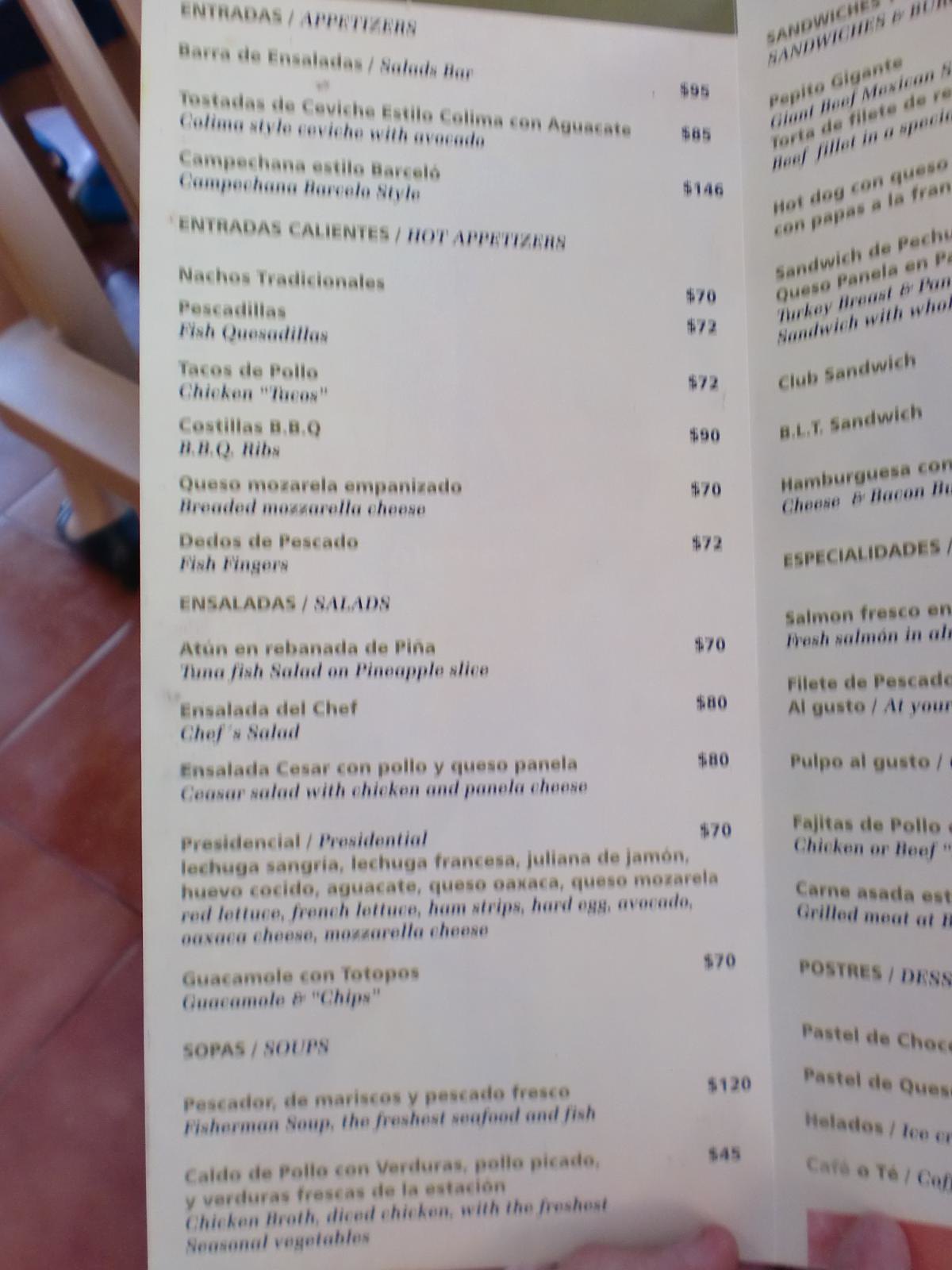This photograph captures a menu from a Mexican restaurant, likely located in Mexico, given that all the prices are listed in pesos. The image is taken in what appears to be a restaurant with a pink floor visible in the background. The bottom of a table and possibly the shadow of someone sitting nearby can also be seen. 

The menu is being held in the lower right corner of the photograph by two thumbs, which are visible in the frame. The menu features multiple main sections, each listed in both Spanish and English. These sections include "Entradas Calientes" (Hot Appetizers), "Ensaladas" (Salads), "Sopas" (Soups), "Sandwiches", and "Especialidades" (Specialties). There is also a section for "Postres" (Desserts). 

Although only one page of the menu is fully visible with the second page partly shown, you can see detailed listings under each heading. For example, fish quesadillas are priced at 72 pesos, tacos de pollo (chicken tacos) are also 72 pesos, and barbecue ribs as an appetizer are 90 pesos. The menu includes a variety of items, appealing to both local patrons and English-speaking tourists.